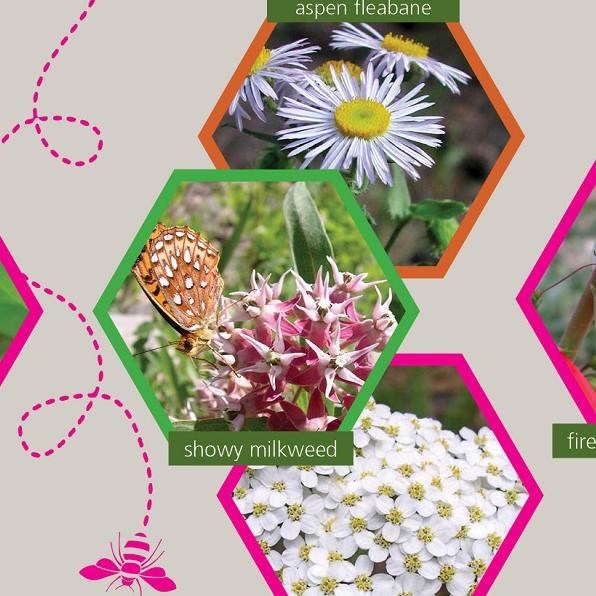The image, likely an advertisement or educational material on a tan background, combines bright splashes of orange, vibrant green, and hot pink. At the left, an illustrated bumblebee traces a playful, dashed loop-de-loop trail across the page, evoking a sense of movement. Central to the image are a series of hexagons resembling a honeycomb, each framing a different wildflower, highlighting the theme of a pollinator-friendly garden. 

The first hexagon on top displays a photograph of aspen fleabane, reminiscent of a delicate daisy with numerous white petals radiating from a yellow center. Below it, a hexagon showcases the showy milkweed, characterized by its spiky pink flowers, and accompanied by a fritillary butterfly perched on a leaf. The lowest hexagon contains a cluster of small, white flowers with yellow centers. These hexagonal frames not only segregate the images but also enhance the thematic connection to bees and pollination. The image is adorned with both photographic and hand-illustrated elements, providing detailed insights into creating a bee-friendly garden.